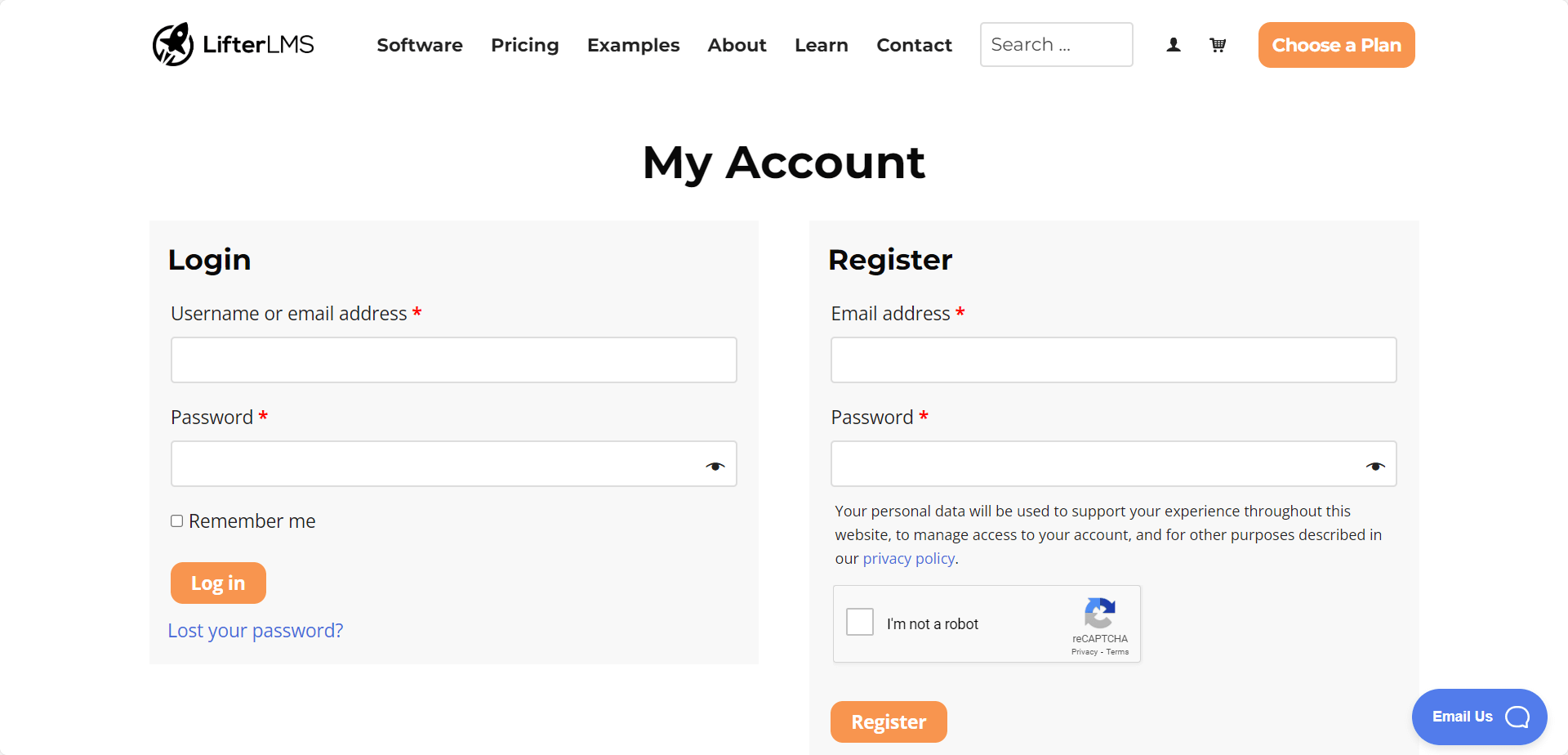This is a screenshot from a website featuring the Lifter LMS platform. At the top left corner in black font, the title "Lifter LMS" is displayed, accompanied by a black icon of a small rocket ship blasting off towards the upper right from a circle. Next to the title is a navigation menu with the following options: "Software," "Pricing," "Examples," "About," "Learn," "Contact," and an integrated search field within a small rectangle.

To the right of the menu, there is a silhouette icon of a man's head followed by a shopping cart icon. Adjacent to these icons is a prominent green button with the text "Choose a Plan" in white font.

Below the header, a large section with bold black text reads "My Account." This section is divided into two gray boxes. The box on the left is for existing users and is labeled "Login." It contains two input fields: one for "Username or Email Address" and another for "Password," both marked with an asterisk indicating required fields. Below these fields, there is a checkbox option labeled "Remember Me." Under the checkbox is a green button labeled "Login," and beneath it, a blue link that reads "Lost your password?"

To the right, the second gray box is labeled "Register." This section includes fields for "Email Address" and "Password," and below these fields, there is a checkbox labeled "I'm not a robot" for CAPTCHA verification.